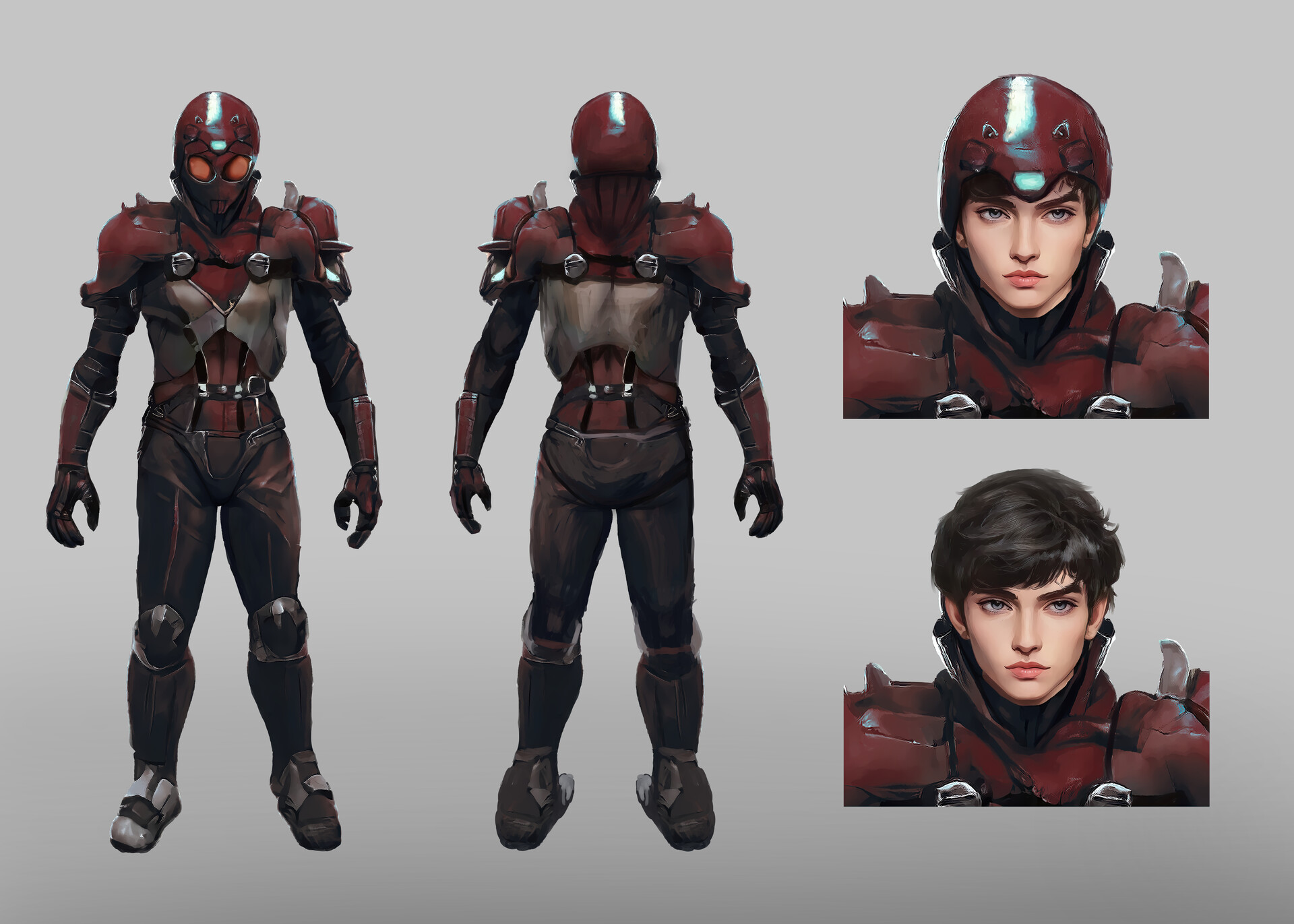The image showcases a video game character in detailed combat gear. On the left side, the character is depicted both from the front and back, wearing a maroon and silver armored suit that covers the entire body, leaving only a narrow opening for the eyes. The front view shows the character facing the camera with a menacing stance, while the back view highlights the elaborate design of the suit. To the right, there are two vertical headshots of the same character. The top headshot features the character wearing a red helmet that partially reveals his face, showing his blue eyes and arched eyebrows. The bottom headshot displays the character without the helmet, revealing his black hair. The character appears to be a young man, likely a teenager or in his early 20s. The gray background emphasizes the stark contrast of the dark, immersive colors and intricate details of the combat gear.